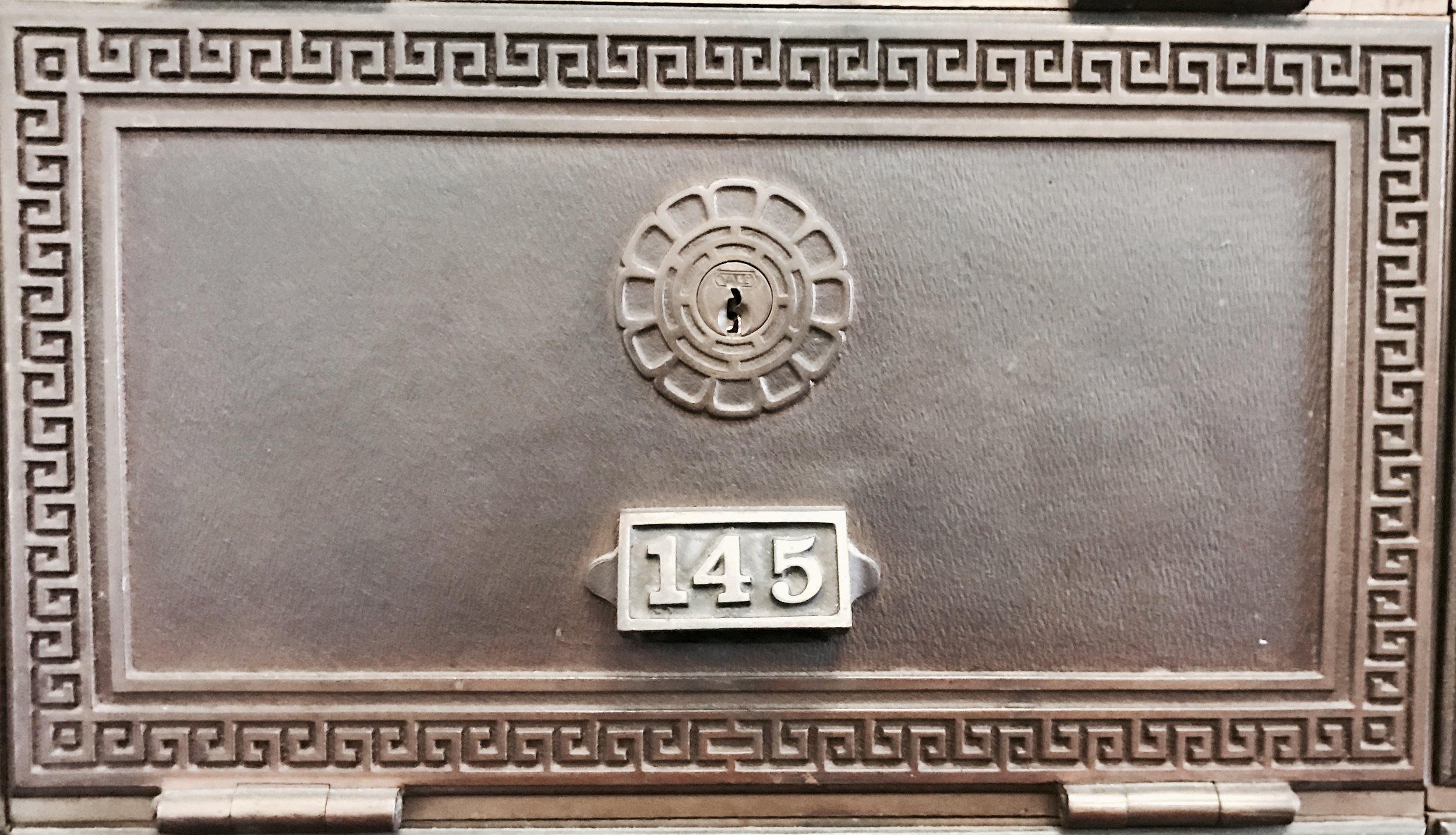The image showcases the face plate of an ornate safety deposit box numbered 145. This metal box, possibly designed between the 1920s and 1960s, is adorned with an intricate, maze-like mosaic border that features raised surfaces and angular tracks. The box has a washed-out, slate gray color with hints of silver, suggesting an antique feel and giving it a muted, sepia-toned appearance. The number 145, located prominently in the middle of the face plate, is slightly illuminated, making it stand out against the otherwise subdued palette. There's an open key slot at the top, indicating where a key would be inserted to unlock the box. The hinges are located at the bottom, suggesting that the door would open downwards, parallel to the ground, allowing access to the contents inside.